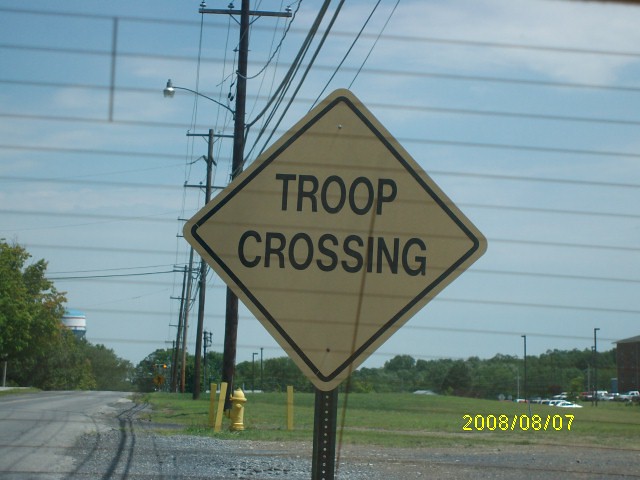The daytime photo, taken from the rear window of a car with visible defrost lines, captures a rural street scene dated 2008-08-07. Dominating the center of the image is a yellow and black diamond-shaped "Troop Crossing" sign, mounted on a post. The landscape features two roads: a gravel road stretches horizontally across the bottom, while a paved road diverges from the bottom left into the distance. The scene includes several power poles with accompanying wires, a street lamp extending from one of the poles, and a yellow fire hydrant directly ahead. In the background, numerous trees populate the horizon, and the top of a water tower is visible to the left amidst the greenery.